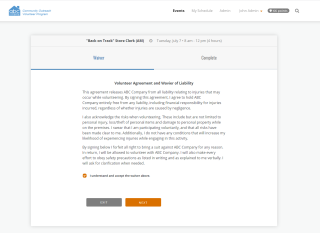The image depicts a website interface. At the top, there is a white banner followed by a blue section, which resembles the outline of a house containing some text that is illegible due to blurriness. Further down, there's light blue text, also unreadable. Below this area, there is darker black text stating "Events" and "My Schedule," though these words are pale and not easily decipherable.

Continuing down, the background shifts to a light gray color. Centrally located, there is a header featuring some difficult-to-read black text at the top. Beneath this, slightly clearer light text indicates event times, reading "Tuesday, July 7th, 8am, 12pm, 4 hours." Following this segment, blue underlined text appears alongside more black text, set against a transitioning white background. This section is titled "Volunteer Agreement," which includes mentions of liability and details about the agreement itself.